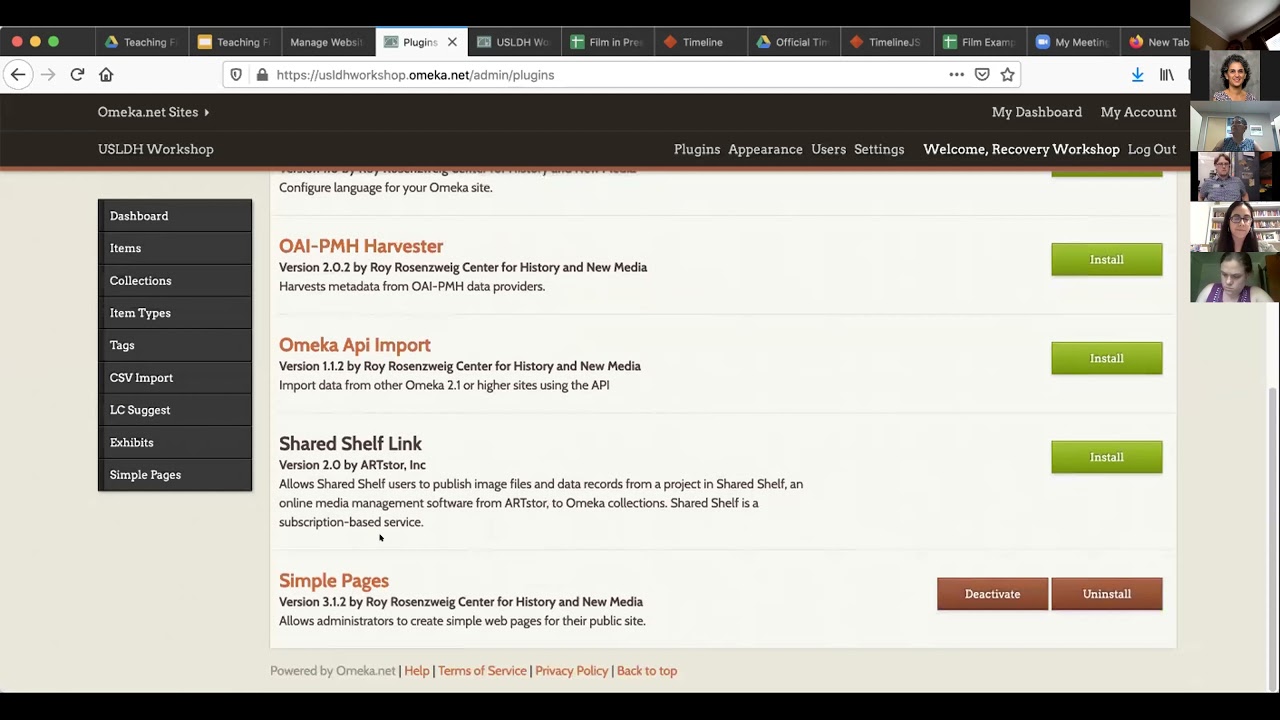The image is a screen capture showcasing a web conference meeting, where five participants' thumbnail images are displayed in the top right corner of the screen. The main content being shared is from an Apple device running the Chrome web browser, evident by the numerous open tabs. The visible tabs hint at the meeting's focus, with names like "teaching," "Google Drive," "research website," "plugins," "USLDH," "film and PRE," "timeline," "official timeline," "film example," "my meeting," and "new tab," indicating a diverse range of topics possibly related to educational content and web management.

The website open in the browser is http://usldhworkshop.omeka.net/admin/plugins, part of the Omeka content management system. The interface prominently features a navigation menu on the right, which includes "omeka.net sites" with an arrow pointing right, "my dashboard," "my account," "USLDH workshop," and options like "plugins," "appearance," "users," "settings," "welcome," "recovery," "workshop," and "log out."

On the left, a vertical menu lists options in white text on black rectangles, including "dashboard," "items," "collections," "item types," "tags," "CSV import," "LC suggests," "exhibits," and "simple pages," suggesting a focus on website content management. Below this menu, a list of items that users can scroll through is visible. Each item is associated with a green rectangle labeled "install," though the top item is partially obscured.

Four plugins are clearly listed:

1. **OAIPMH harvester, version 2.02** by Roy Rosenzweig Center for History and New Media: Facilitates harvesting metadata from OAI-PMH data providers.
   
2. **Omeka API import, version 1.1.2** by Roy Rosenzweig Center for History and New Media: Enables data import from other Omeka 2.1 or higher sites via the API.
   
3. **Shared shelf link, version 2.0** by ArtStore Incorporated: Allows Shared Shelf users to publish image files and data records from Shared Shelf to Omeka collections, conditions on subscription-based service.
   
4. **Simple pages, version 3.1.2** by Roy Rosenzweig Center for History and New Media: Permits administrators to create simple web pages for their public site.

Additional controls at the end of each plugin description, which are medium brown rectangles with white text, offer options to "deactivate" or "uninstall" the plugins. At the bottom of the screen, there is a footer stating "powered by Omeka.net" in white text, accompanied by orange links for "help," "terms of service," "privacy policy," and "back to top."

This detailed setup hints that the web conference is focusing on the discussion of suitable plugins for enhancing a website's functionality, particularly within the Omeka platform, which is often utilized for cultural heritage projects.